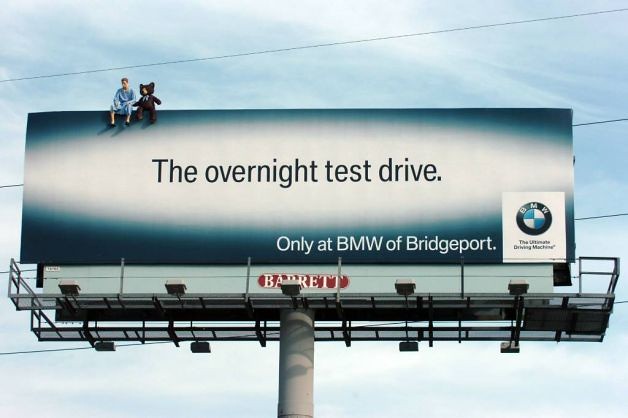The image captures a billboard set against a hazy, light blue sky dotted with cloud cover. The billboard is mounted high on a concrete or possibly metal pillar, equipped with walkways on either side and five floodlights aimed at the sign. Four power lines run above and behind it. The billboard features a design with a dark blue background that transitions into a white oval in the center. The main text in dark letters within the white oval reads "The Overnight Test Drive," while additional text on the blue background at the bottom states, "Only at BMW of Bridgeport." In the bottom right corner is the BMW logo, consisting of a circle divided into blue and white quadrants, with the letters BMW at the top and the slogan "The Ultimate Driving Machine" underneath. At the top left corner of the billboard, there appears to be a depiction of a man in long-sleeve pajamas sitting next to a teddy bear, both facing us. The billboard belongs to the company Barrett, as indicated by their name partially visible. The perspective of the photograph is angled from below, accentuating the height and structure of the billboard.